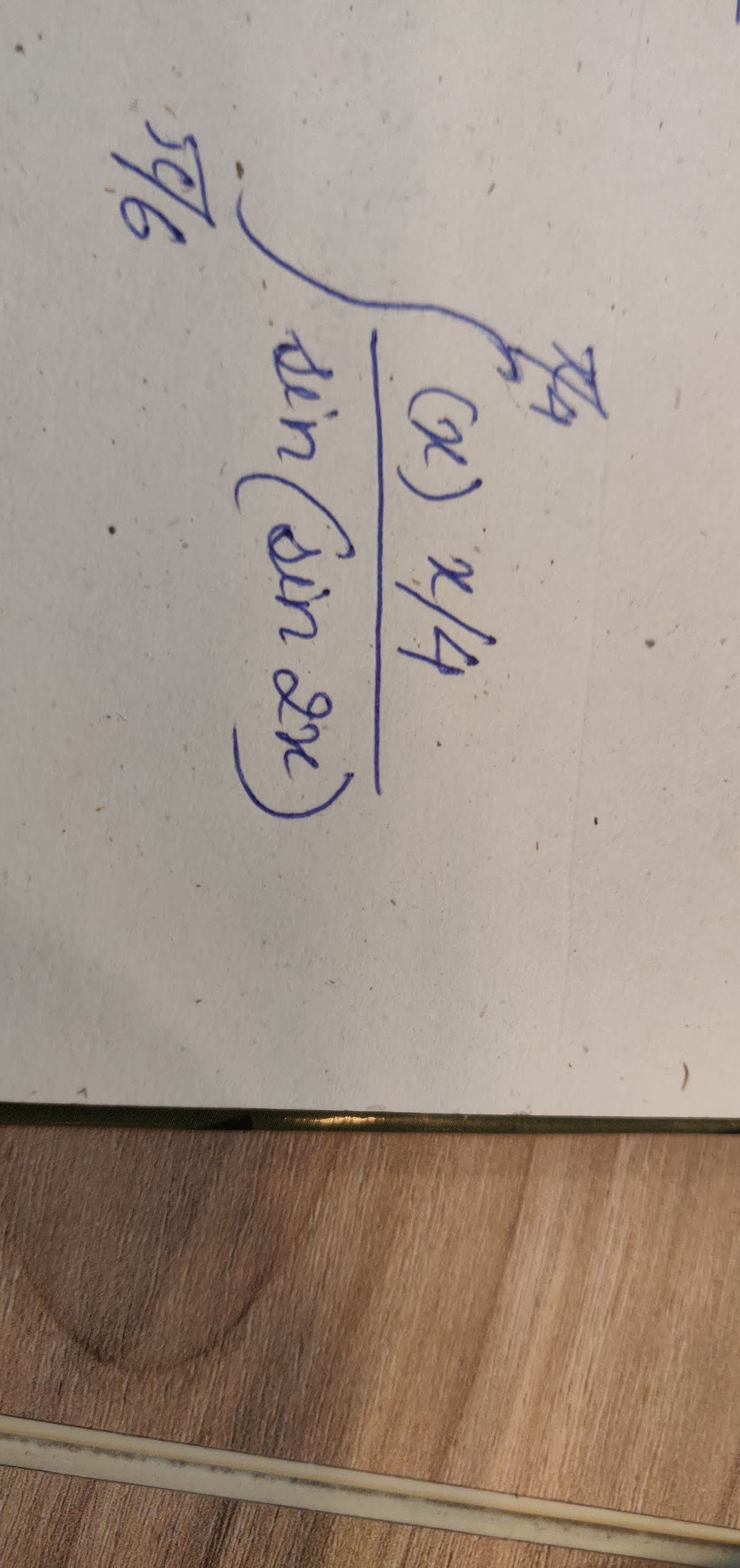A piece of white paper, positioned sideways on a light brown wood grain table, features blue ink markings that appear to be a mathematical equation. The equation begins with bracketed variables, potentially written as [x] x/4. Below this, a line separates the initial expression from what seems to be 'sin(2x)', indicating a trigonometric function. Towards the middle of the equation, a long, somewhat ambiguous squiggle resembles an 's' shape, with a number '6' discernible at its base. Additionally, more squiggles near the top hint at angular geometric shapes, possibly resembling portions of a triangle. However, the equation remains incomplete, with no final answer provided within the image.